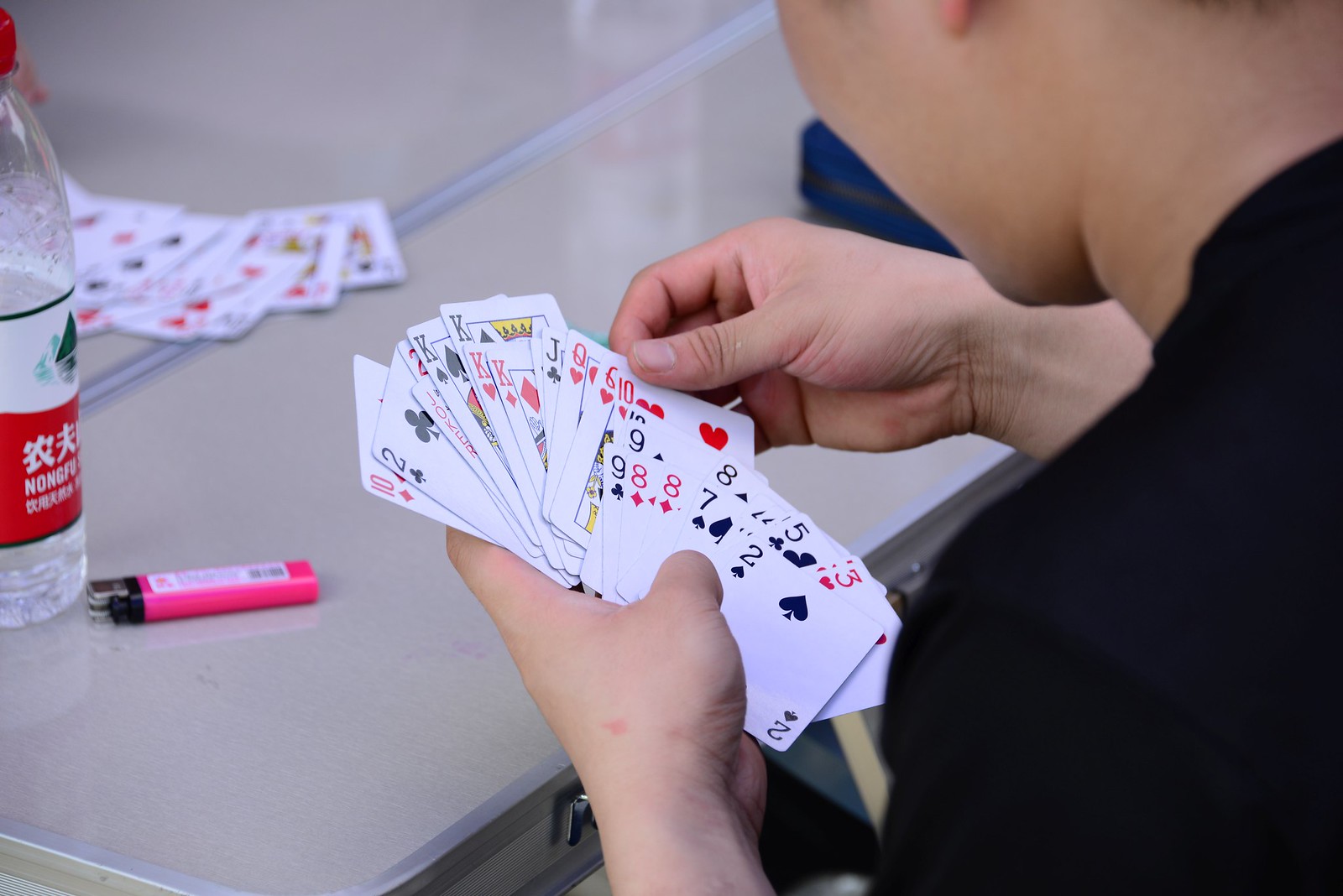In this image, a person is engrossed in a card game, likely not in a typical lunchroom setting despite initial impressions. The scene is set at a clean, white table, adorned with a bright hot pink lighter and a notable Nongfu Spring water bottle, identifiable by its red and white label and red cap with Asian text. The player, dressed in a black t-shirt, faces away from the camera, revealing the intricate layout of their hands. Their cards, meticulously displayed from left to right, include: 10 of diamonds, 2 of clubs, a red 2, a joker, king of spades, another king of spades, king of hearts, king of diamonds, an obscured card, jack of clubs, queen of hearts, another queen of hearts, 10 of hearts, an unidentified black 10, 9 of spades, 9 of clubs, 8 of diamonds, another 8 of diamonds, 8 of spades, 7 of spades, two black 4s, 5 of clubs, 3 of hearts, another 3 of hearts, and 2 of spades. A blurred pile of cards lies in the center of the table, hinting at an ongoing game with visible face cards and a faint glimpse of another player's hand behind the water bottle, suggesting active card discarding into the central pile.